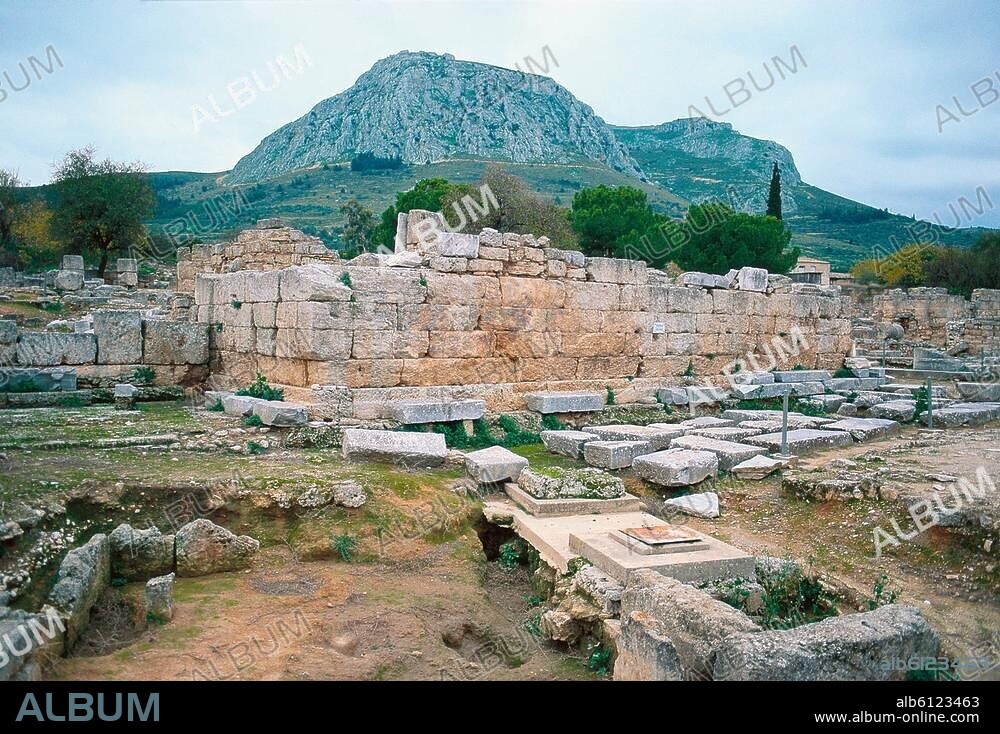The image displays a scenic view, prominently watermarked with the word "album" in grey diagonal text across it and features a black rectangular strip at the bottom bearing the white text "album" on the left, alongside "ALB6123463" and "www.album-online.com" on the right. The background is graced with a vivid blue sky above rugged, rocky mountains and verdant vegetation, including possibly cypress and ash trees. A central feature is a rustic, brownish-orange stone wall or barrier composed of large rectangular rocks, hinting at an ancient structure or ruin, possibly from Greek, Turkish, or Italian origins. The mid-ground reveals additional wisps of stone remains, perhaps the base of a building with one to four layers of bricks still intact, suggesting a scene of previous archaeological exploration. The foreground is littered with similar large stone blocks yet to be assembled. The photograph encapsulates a blend of history and nature, evoking an archaeological dig site under a bright and clear daytime sky.